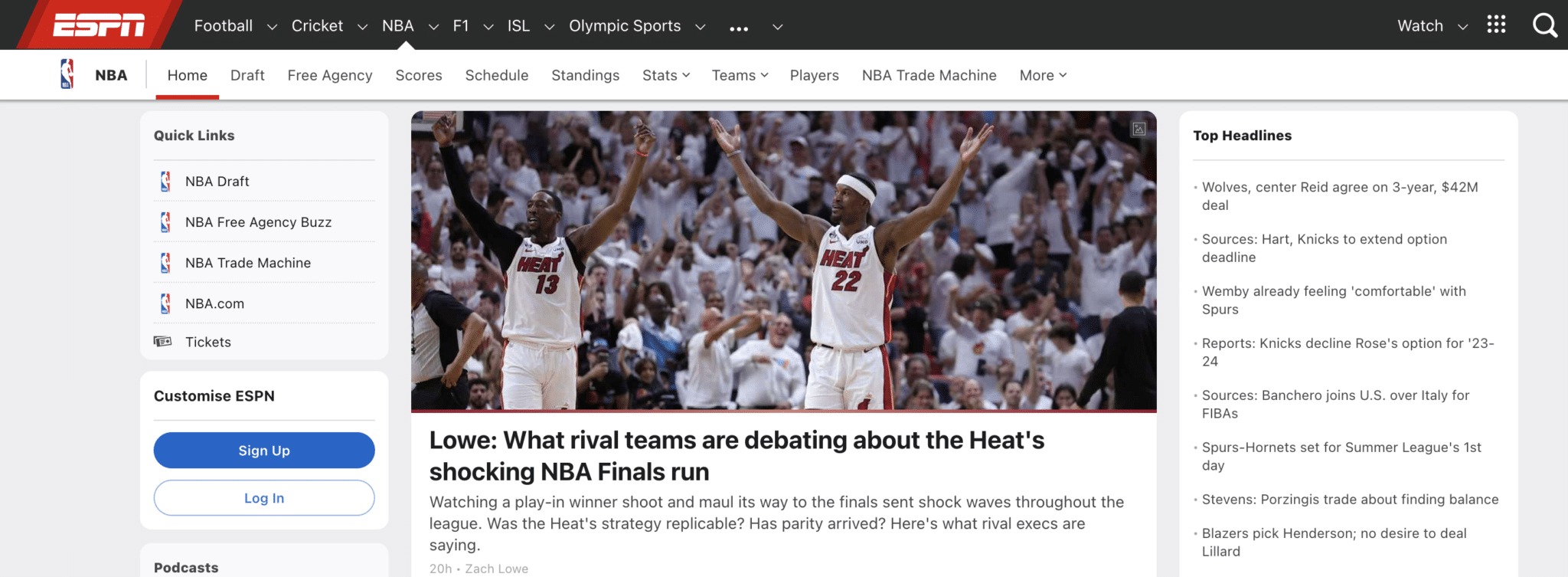This left-to-right horizontal image is a cropped screenshot taken from the ESPN webpage, likely from a computer or smart device. The top of the image features a prominent black rectangular navigation bar with a red background and the white ESPN logo. Adjacent to the logo, menu items like "Football," "Cricket," "NBA," "F1," "ISL," and "Olympic Sports" are listed, followed by an ellipsis indicating more options. On the top right corner, the navigation bar includes items labeled "Watch," a grid icon consisting of nine small circles, and a magnifying glass icon indicating search functionality.

Below this navigation bar, towards the left beneath the ESPN logo, an NBA section is visible. This section includes links such as "Home," "Draft," "Free Agency," "Scores," "Schedule," "Standings," "Stats," "Teams," "Players," "NBA Trade Machine," and "More." The "Home" link is highlighted with a red underline, suggesting it is the selected option. Directly underneath "Home," quick links like "NBA Draft," "NBA Free Agency Buzz," "NBA Trade Machine," and "NBA.com Tickets" are available, along with prompts to customize ESPN by signing up or logging in. There is a mention of "Podcasts" below, though the rest of the word or section is cut off in the image.

The central portion of the screenshot features a picture of two Miami Heat players accompanying an article titled, "What rival teams are debating about the Heat's shocking NBA finals run." A short blurb about the article is also partially visible.

On the upper right side of the image, a "Top Headlines" section is noted, with "Top Headlines" bolded. Below this, a list of clickable storylines is present, though the specifics are obscured due to cropping. The overall image captures the essence of the ESPN webpage, highlighting its organized layout and content focus on NBA updates and major sports headlines.